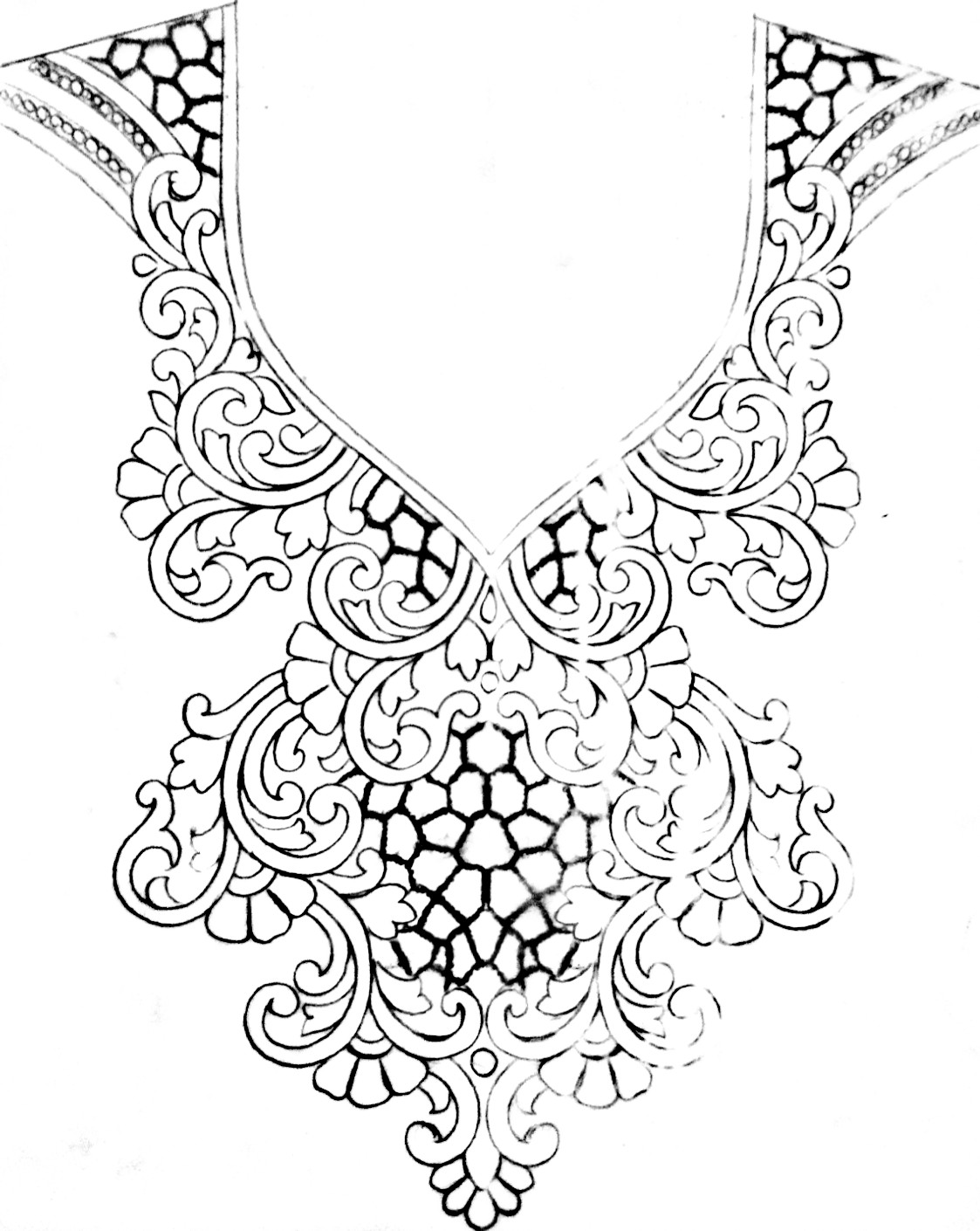The image displays a meticulously detailed, hand-drawn sketch of a corset set against a pure white background. The corset is illustrated in black ink, emphasizing both pattern and structure. Its design is heavily adorned with floral and scroll motifs along the edges, creating an intricate and ornate appearance. The corset has a deep sweetheart neckline that transitions into a V-shape, enhancing the hourglass figure before reaching the shoulders where the lines become parallel. The central area of the corset is filled with a complex tiling pattern, adding to its elaborate aesthetic. The design gives an impression of curvature at the hips, suggesting a fitted silhouette. The combination of these elements evokes the delicate craftsmanship of lace or wrought iron work, blending the elegance of a designer garment with the detail of intricate wire art.